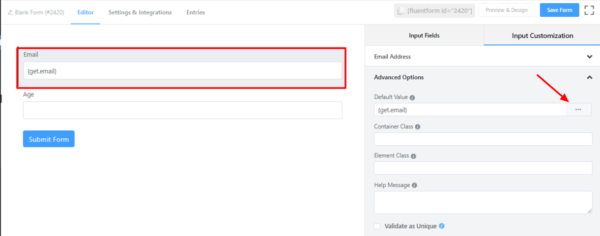The image displays a blurred screen capture, likely taken from a laptop or desktop monitor, given its rectangular shape. In the top-left corner, there is some gray lettering that is illegible due to the blur. To the right, the word "Editor" appears in dark blue, followed by "Settings" in black and some additional, unreadable text in gray.

Currently, the "Editor" tab is selected. Below it, on an off-white background, there is a red, bold-outlined rectangle filled with a gray interior, labeled "Email" in black. Beneath this rectangle is a white input bar that contains the placeholder text: "| get email |". Further down, there is another input field labeled "Age."

In the bottom left corner, a blue button with white text reads "Submit Forms." On the right-hand side of the screen, the top section contains illegible text that seems to include the word "Save." Below this, two categories are listed on a gray background: "Input Fields" and "Input Customization." These categories are more legible and include alternating white and gray options: "Email Address," "Advanced Options," "Default Value," "Container Class," "Element Class," and "Help Message." Additionally, there is a radio button labeled "Validate as Unique" with a blue information icon next to it.